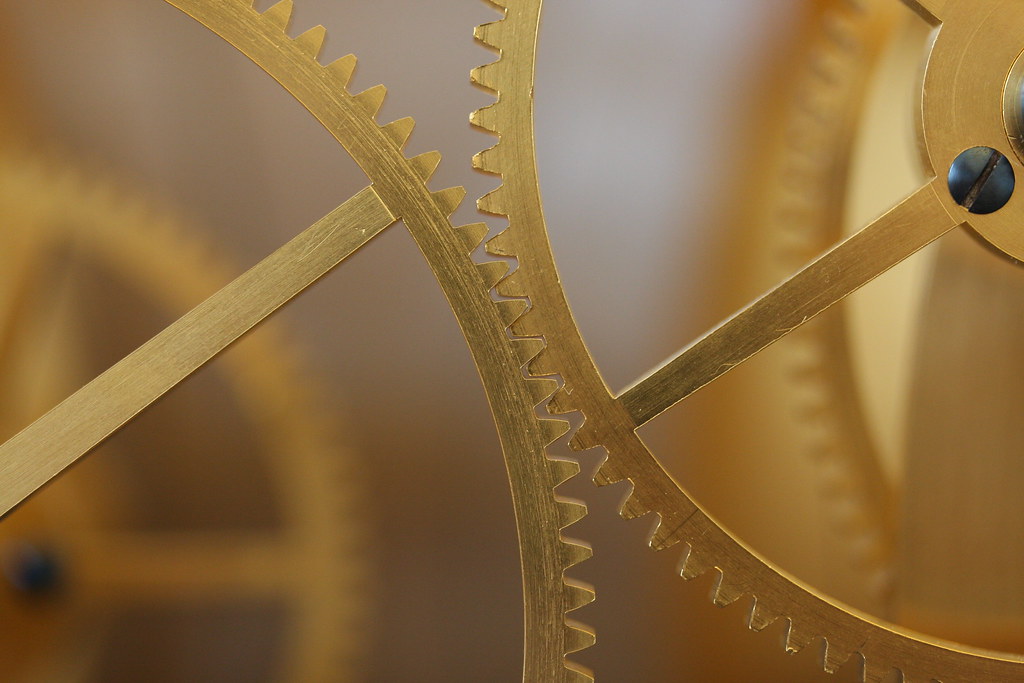This image is a precisely focused close-up of two brass-colored gears with meshing teeth. The photo highlights the connection between the gear teeth, making them the central focus while the background fades into a blur, rendering other gears barely distinguishable. Both gears are designed with spokes, extending from a central connector towards their teeth. On the right-side gear, there's a notable black flathead screw just within the frame, though the gear's center lies just beyond the focus area. In contrast, the left-side gear only reveals part of a spoke. The overall composition emphasizes the detailed meshing of the gears' teeth, creating a striking contrast with the indistinct, grayish-white blurred background.